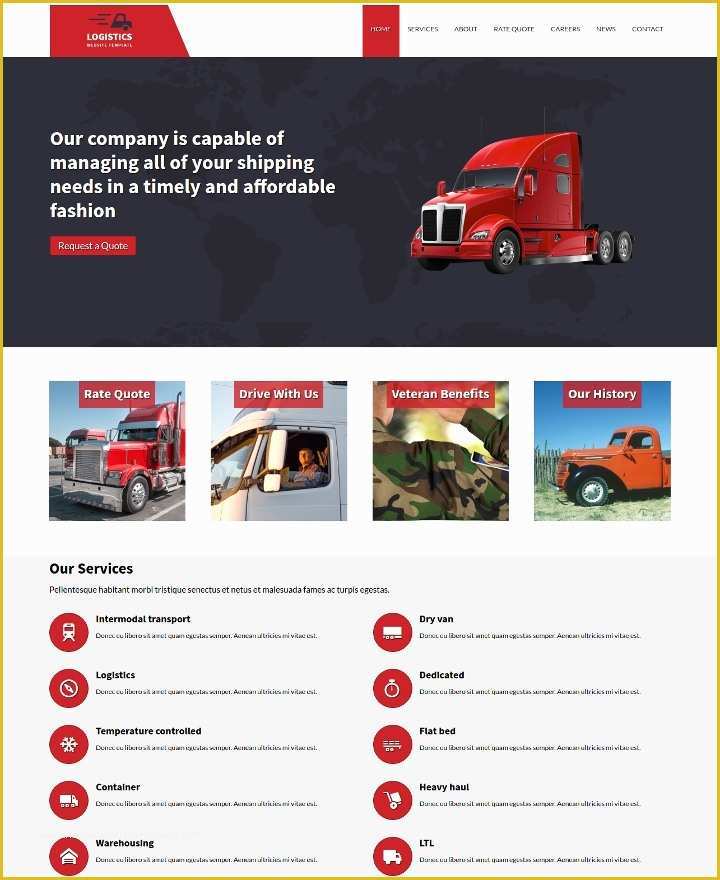This is a screenshot of a website named "Logistics." The logo, positioned on the top left, features a cartoon image of a truck with three horizontal lines beside it, suggesting motion. The company's name, "Logistics," is displayed in bold, white font with smaller text beneath it.

To the right of the logo is a navigation menu with tabs labeled: Home, Services, About, Rate Quote, Careers, News, and Contact. The "Home" tab is highlighted in a red square, indicating the current page.

Dominating the upper section of the page is a large gray banner. The background of this banner is a subtly faded world map, overlaid by an image of a red truck on the right side. The banner includes the text: "Our company is capable of managing all your shipping needs in a timely and affordable fashion," and beneath this, a button labeled "Request a Quote."

Below the banner, the page presents four clickable images, each representing different sections of the site:
1. "Rate Quote" with an image of a red truck.
2. "Drive with Us" featuring a man driving a truck.
3. "Veteran Benefits" showing a man in camouflage saluting.
4. "Our History" displaying an orange-red truck parked outside.

At the bottom of the page, several service options are listed with corresponding icons. These include Intermodal Transport, Logistics, Temperature-Controlled Shipping, Container Shipping, Flatbed Transport, Dedicated Services, and Dry Van Shipping, representing the various services offered by the company.